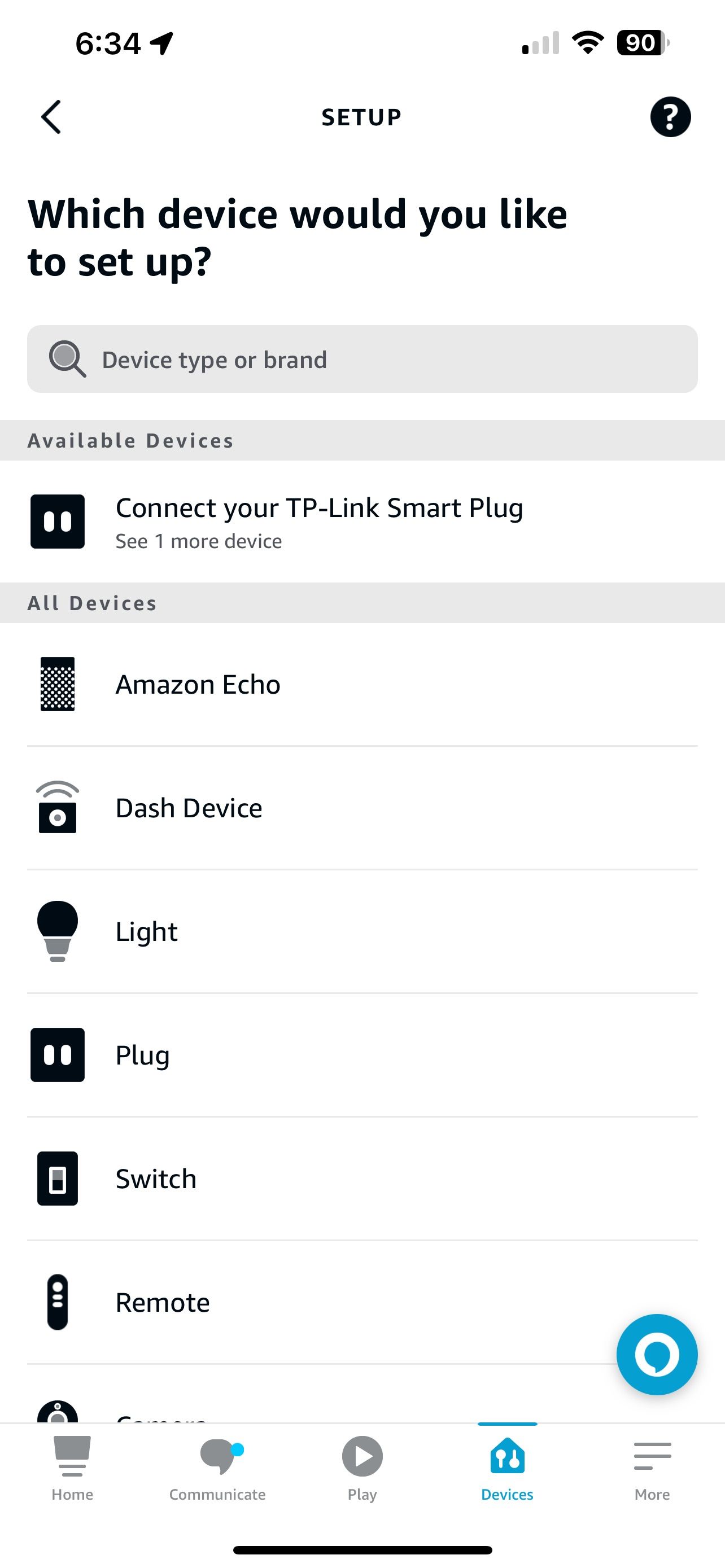In this image, we see a screenshot from a smartphone displaying a setup page for connecting devices. The page features a variety of options laid out in a detailed list. At the top, the page asks, "Which device would you like to set up?" and includes a search bar with placeholder text saying "device type or brand," alongside a magnifying glass icon for searching.

Below this prompt, there is a section for available devices, of which there is currently one listed: "Connect your TP-Link smart plug." There's a note indicating "see one more device," suggesting a second available device may be present but not immediately displayed.

The majority of the page showcases a comprehensive list of all supported devices. This list includes:
1. Amazon Echo
2. Dash device
3. Light
4. Plug
5. Switch
6. Remote
7. A partially visible option that appears to be a camera

Each device type is accompanied by an icon representing its function, all depicted in a monochromatic color scheme, lending the page a clean, minimalistic appearance.